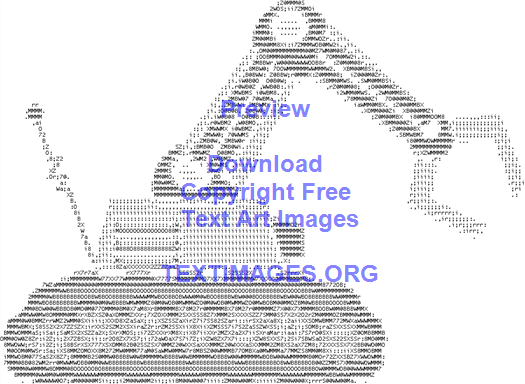The image presents a stock advertisement for a text art website showcasing copyright-free text art images from TextImages.org. Dominated by a plain white background, the centerpiece is a pixelated, grayscale representation of a robotic machine, reminiscent of the output from a dot matrix printer. This artwork, crafted entirely from keyboard characters and numbers, exhibits a machine featuring a large tank-like track at its base, a bent arm extending forward, and a wrench-like claw directed to the right. An antenna with a ball on top protrudes from the machine's rear. Overlaid in purplish-blue text are the words: "Preview Download Copyright-Free Text Art Images" followed by "TEXTIMAGES.ORG" in all caps. The simplicity of the image, combined with its retro, computer-generated aesthetic, highlights the intricate detail possible through text-based art.